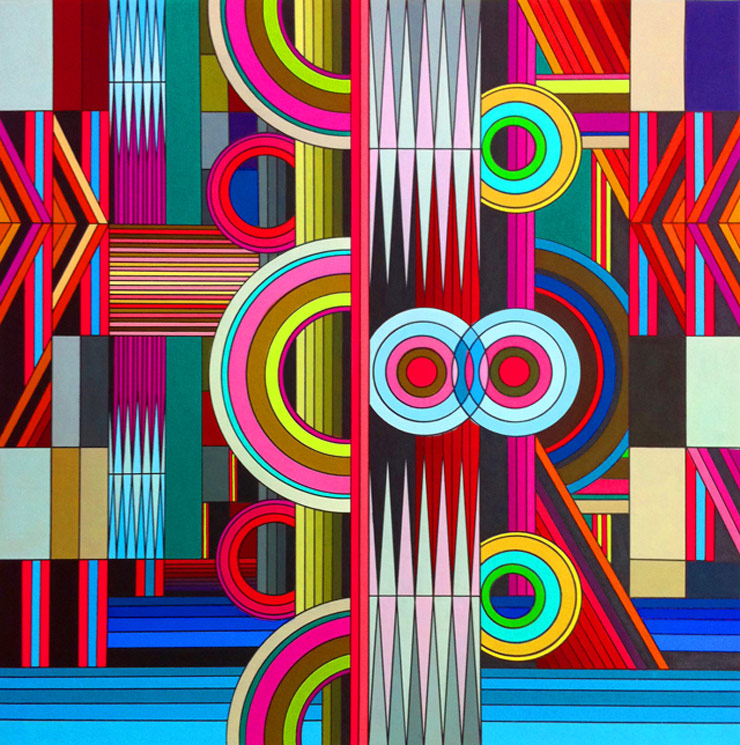The image showcases a vibrant, 1970s-inspired geometric design. Dominating the center is a tall rectangle adorned with intricate white, black, and red diamond patterns. Surrounding the central rectangle are a myriad of shapes, including an array of colorful triangles and squares with parallel lines on either side. Encircling and layered behind this focal point are multiple rows of circles, each varying in color and arrangement. Some circles are translucent, revealing intersecting lines and colored rectangles beneath them, creating intricate overlaps and new color blends. The entire composition is a rich tapestry of intersecting shapes and hues, epitomizing a retro, geometric aesthetic.